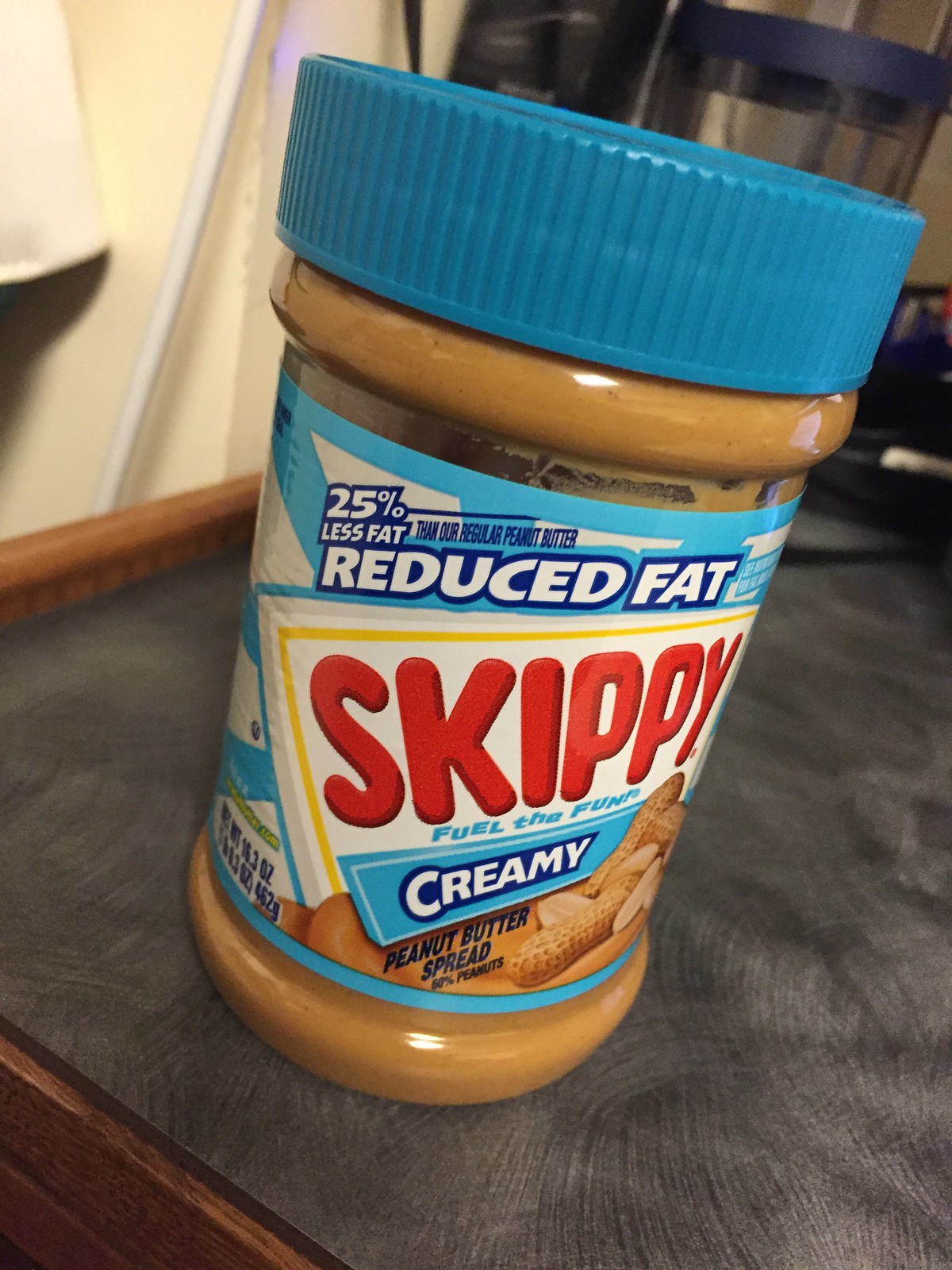The image features a jar of Skippy brand peanut butter prominently displayed. The label on the jar is visually striking, with the word "Skippy" written in bold red letters against a white, rectangular background that is bordered by a thin yellow line. Directly below the brand name is the slogan "Fuel the Fun" printed in blue. Beneath this slogan, a blue rectangle contains the word "Creamy," indicating the texture of the peanut butter. At the very top of the label, the jar boasts "25% Less Fat" and "Reduced Fat" in small blue and white text, clarifying that this variety has less fat than Skippy's regular peanut butter. The bottom part of the label identifies the product as a "Peanut Butter Spread," and displays some peanuts on the right-hand side.

The background of the label features radiating blue lines, adding a dynamic feel to the overall design. The jar itself is capped with a blue lid, allowing a glimpse of the creamy peanut butter inside.

The setting is cozy and slightly rustic; the jar rests on a black, textured surface with a wooden frame surrounding it. In the top-left corner, there's a yellowish wall contrasted by a white pole. Behind the jar, you can spot some black kitchen appliances and a partially see-through item along with a white object, providing a homely backdrop.